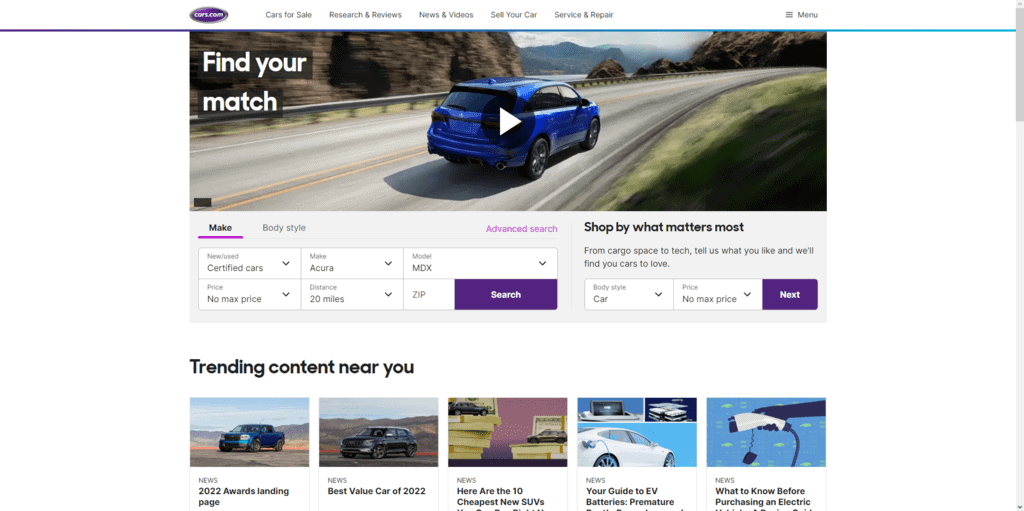This screenshot captures the homepage of the website "Cars.com". At the top, there's a prominently displayed logo that reads "cars.com" in white text within a purple oval. The navigation bar below the logo includes several categories: "Cars for Sale," "Research & Reviews," "News & Videos," "Sell Your Car," "Service & Repair," and a "Menu" button positioned on the far right.

Just below the navigation bar, there is a large video section with the title "Find Your Match." The still frame of the video shows a blue car driving down a scenic mountain road, with a body of water visible in the background. A play button is centered on the image, inviting users to watch the video.

Underneath the video, there are a series of dropdown menus designed to help users search for cars. The currently highlighted dropdown is "Make," and other available options include "Certified Cars," "No Max Price," "Make," "Distance," "Model," and "Zip." A large purple "Search" button is located next to these menus. Additional search options are available under categories like "Body Style," accompanied by the text: "Shop by what matters most from cargo space to tech. Tell us what you like and we’ll find cars to love." This section includes two dropdown menus for "Body Style" and "Price," followed by a "Next" button.

At the bottom of the page, five image thumbnails represent different stories. Three of these images feature cars, one shows stacked piles of money with cars parked on top, and the final image is unclear. The stories are titled from left to right: "2022 Awards Landing Page," "Best Value Car of 2022," "Here Are the 10 Cheapest New SUVs," "Your Guide to EV Batteries," and "What to Know Before Purchasing an Electric Vehicle."